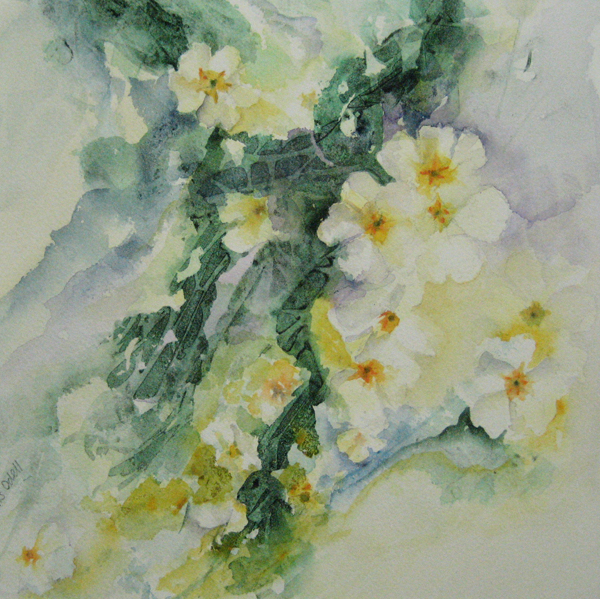This watercolor painting presents an intricate composition of vibrant flowers and lush foliage against a marbled background. Dominating the scene are wide-open, large blossoms with six or more delicate petals in shades of light yellow, resembling cherry blossoms. Their centers boast a vivid yellow hue accompanied by subtle strands of orange. These flowers grow in clusters along multiple tall stems that rise prominently from the bottom to the top of the canvas, surrounded by deep green leaves with undertones of bluish or purplish hues.

The background interplays with varying shades of blue, black, and cream, interspersed with occasional ribbons of yellow that streak across the lower section. Hints of purple and white add depth and suggest an almost ethereal quality. The entire piece, encased within a square frame, gives off a soft, almost blurry effect characteristic of watercolor, making the overall impression both mesmerizing and beautifully nuanced. The flowers and greenery drift towards the top right corner, expanding outwards, adding a sense of movement and life to the artwork.